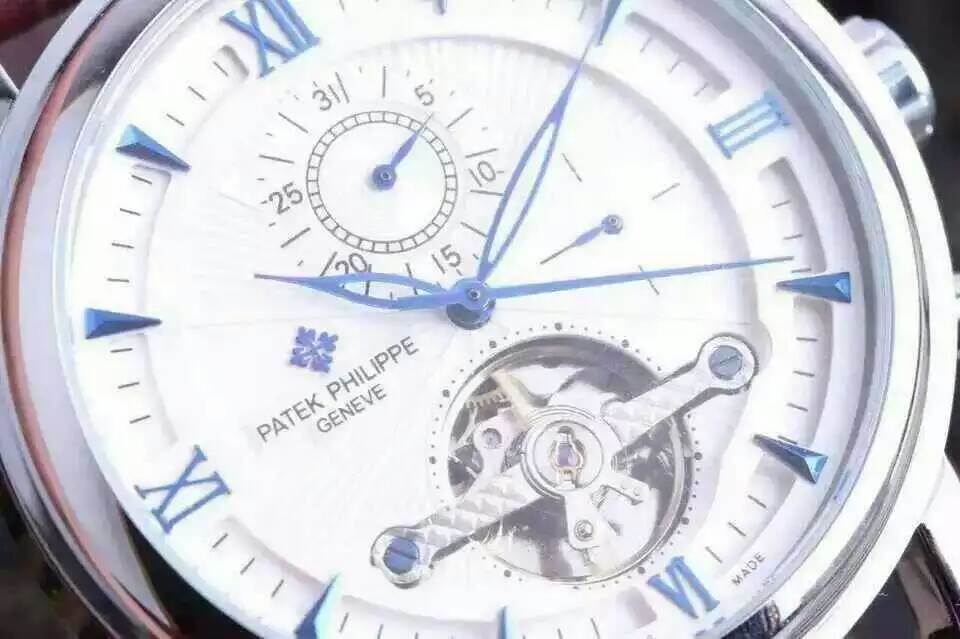This close-up photograph captures the intricate details of a Patek Philippe Geneve watch face. The watch has a white face surrounded by a silver outer edge and features striking blue elements. The timepiece displays Roman numerals - 12, 3, 6, and 9 - in a raised, three-dimensional style, alongside blue triangular markers for the remaining hours. The watch hands are uniquely designed, with the hour and minute hands resembling open ovals tapering to a point, complemented by a long, slender blue second hand. Positioned at the top of the face is a smaller circular dial indicating numbers from 5 to 30. An exposed circular window reveals the watch's intricate inner gears, adding depth and complexity to the design. The silver winding stem is visible at the upper right corner, and the face prominently features the inscription "Patek Philippe Geneve" on the left side. Additionally, the watch is set to 10 past 10, a classic display position.